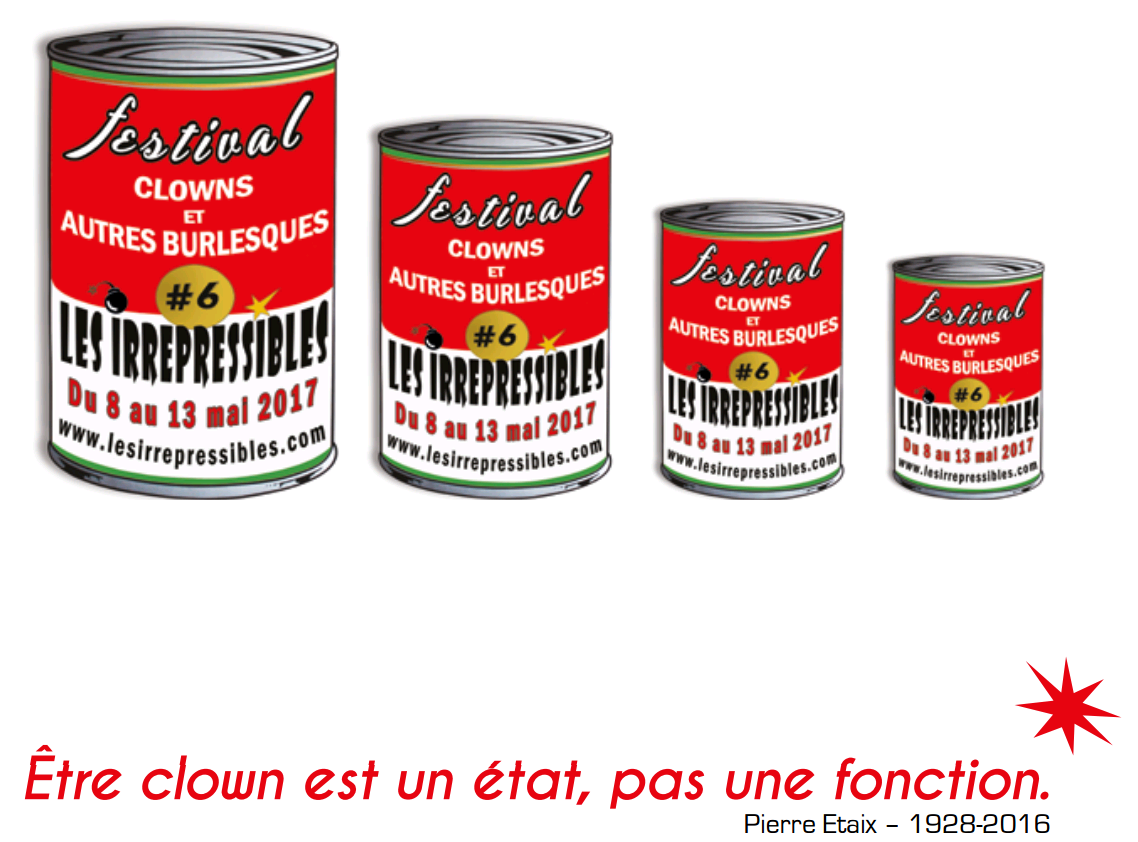The image is an advertisement stylized as a parody of Andy Warhol's soup cans, rendered in a cartoonish style. It features four metallic silver cans with the iconic red and white label reminiscent of Campbell's soup cans. The cans are arranged in a row, decreasing in size from left to right. Each can prominently features the text "Festival Clowns et Arts Burlesques," followed by "Les Irrésistibles," and the date range "8 à 13 Mai 2017." The identical lettering on each can also includes the website "www.lesirresistibles.com."

Beneath the cans, there's a quote in French by Pierre États (1928-2016), which reads, "Être clown est un état, pas une fonction." The image's background is white, putting a strong emphasis on the vibrant colors of the cans and the text, suggesting it promotes a comedy event or group, likely called "Les Irrésistibles." Notably, a small round gold emblem with the number six, a bomb illustration, and a gold star adorn the labels, adding a unique touch to the overall design.